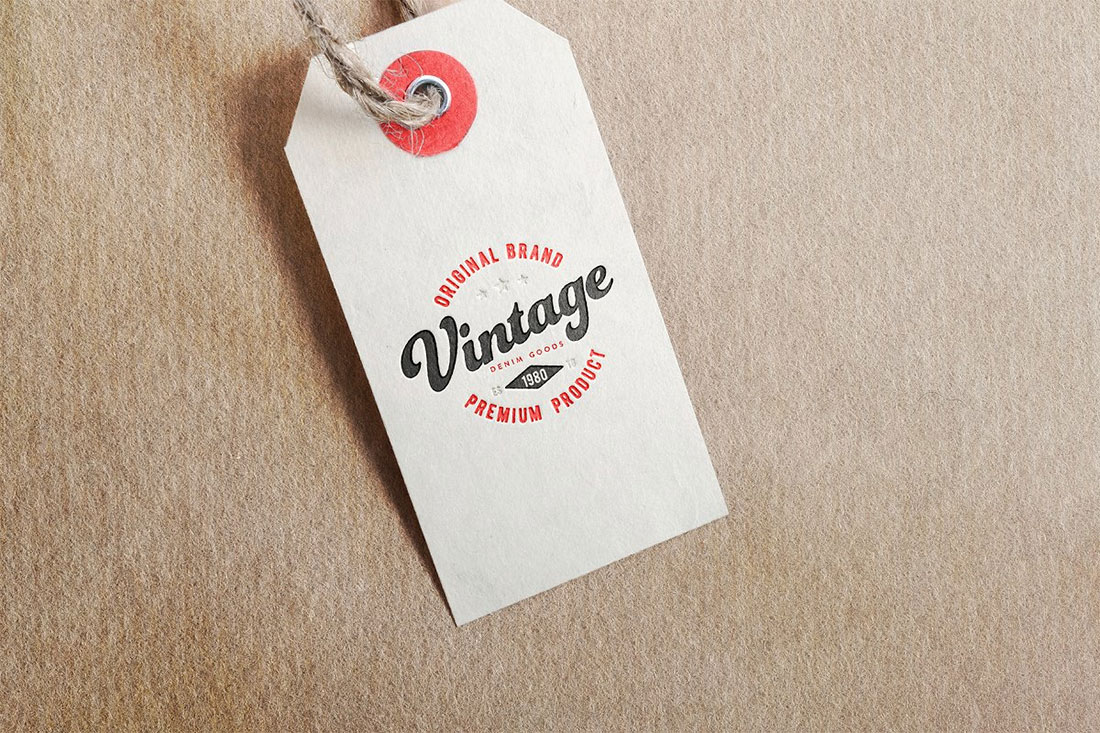This image features a detailed, vintage-inspired tag likely from a pair of jeans. The tag is rectangular with ends cut at an angle, creating a triangular top. Made of white paper, it is set against a textured tan background resembling cardboard or a brown paper bag, possibly like those from grocery stores. The tag's reinforced hole, surrounded by a red circle and a metal grommet, has a burlap or thin twine rope threaded through it for attachment. The text is prominently displayed: "Original Brand" and "Premium Product" are in red, all caps, and form a semicircular pattern around the largest word, "Vintage," which is in bold, semi-cursive script. Below this, "Denim Goods" appears in small red font, and the date "1980" is set inside a diamond-shaped black patch, all centered on the tag. The tag is positioned at about a 45-degree counterclockwise angle across the image, giving it a dynamic layout.